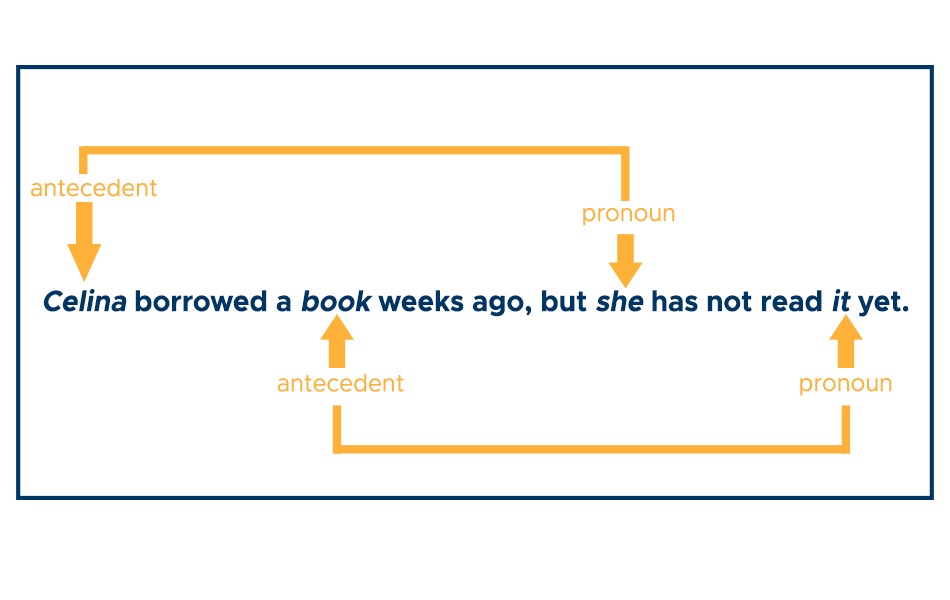This image is a detailed diagram from an English grammar book, illustrating a sentence structure focused on pronouns and their antecedents. The sentence reads, "Selena borrowed a book weeks ago, but she has not read it yet." It features arrows pointing to different parts of the sentence, highlighting the antecedents and pronouns: "Selena," which is the antecedent to "she," and "book," which is the antecedent to "it." The diagram is set against a white background, with the sentence in navy blue and the diagram annotations in orange. The layout is horizontal, clearly delineating each component of the grammatical lesson.